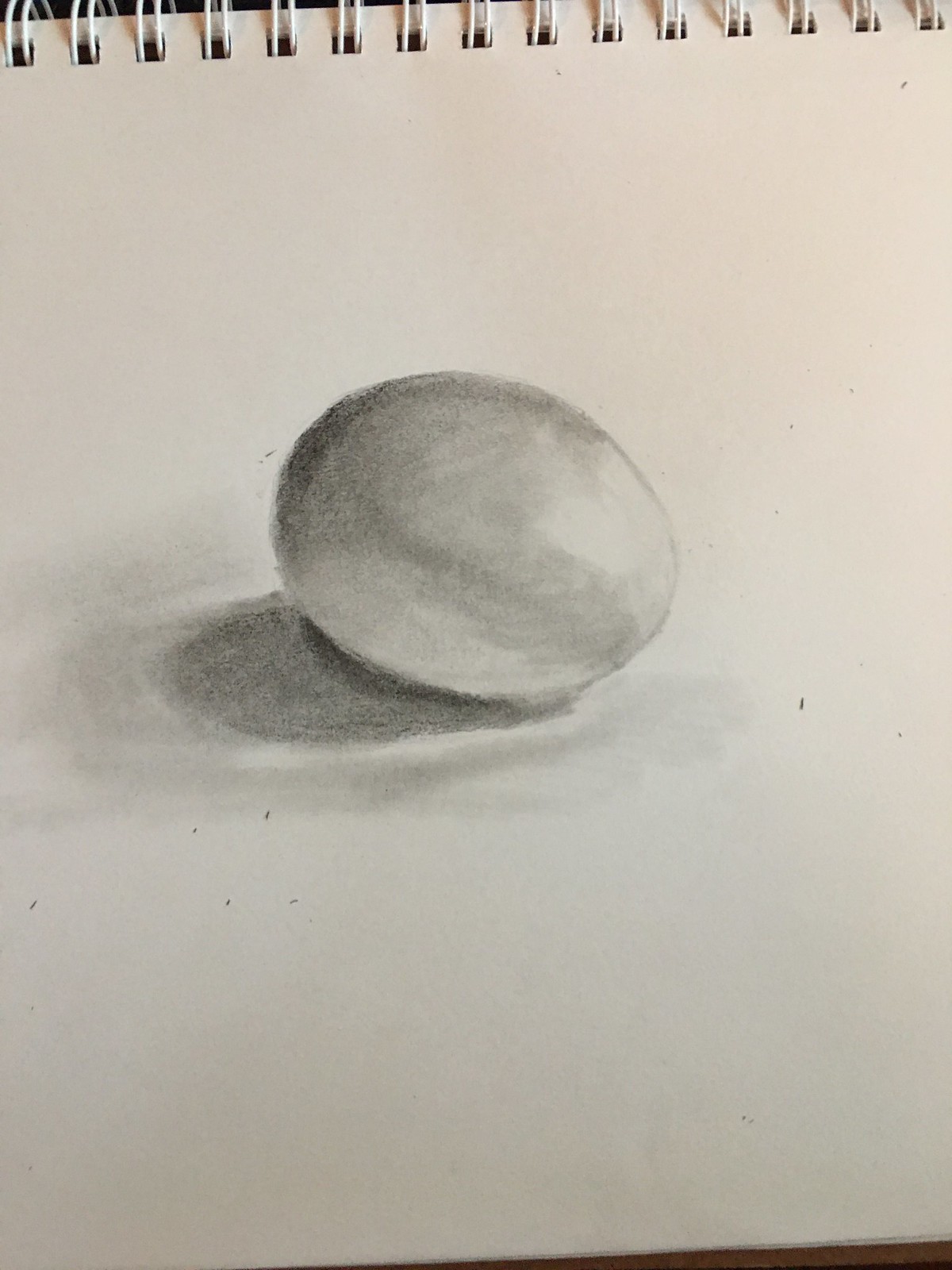This is a portrait-oriented image featuring a meticulously crafted sketch of a 3D sphere. The sphere is expertly shaded, with darker gradients towards the top left, gradually transitioning to lighter, almost white shading towards the bottom right, creating a convincing illusion of depth and dimension. Beneath the sphere, there is a shaded area, darker in tone, suggesting the sphere's recent movement and an impression similar to grass or a textured surface. The background is completely white, providing a stark contrast that makes the sphere stand out prominently. At the top of the image, white ring-like binding structures are visible, holding together multiple pages, implying the sketch is part of a bound sketchbook.